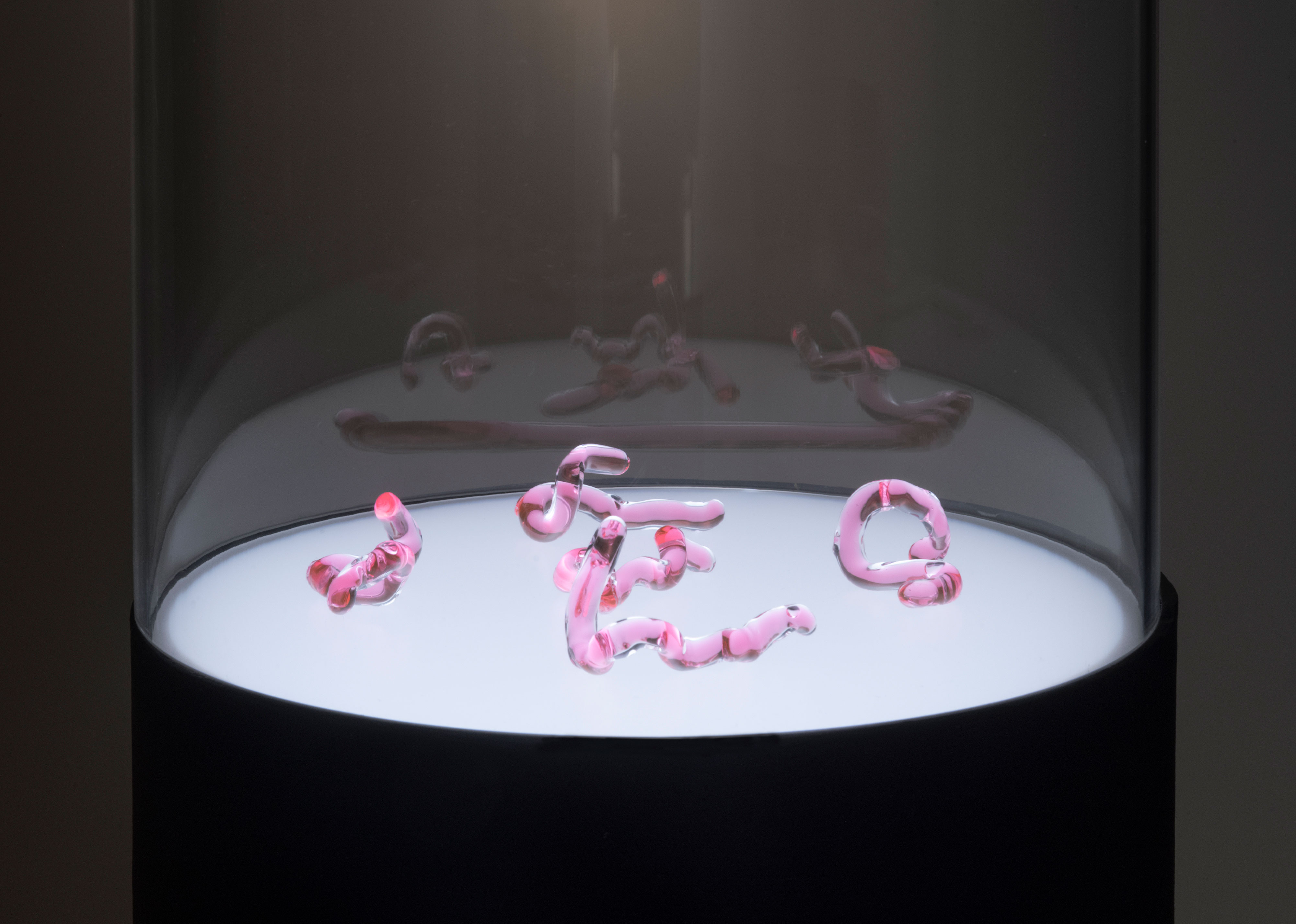The photograph appears to be taken in a lab or scientific setting and features an object prominently centered against a dark gray or black background. The object is a cylindrical jar with a black base and a clear top, possibly made of glass or plastic. Inside the jar, there is a flat, white bottom surface. Arranged on this surface are four pink, tube-like structures that resemble worms, although they are likely made of plastic. These pink objects are contorted into various shapes and their reflections are visible on the clear sides of the jar. The background appears seamless and dark, further emphasizing the jar and its contents.